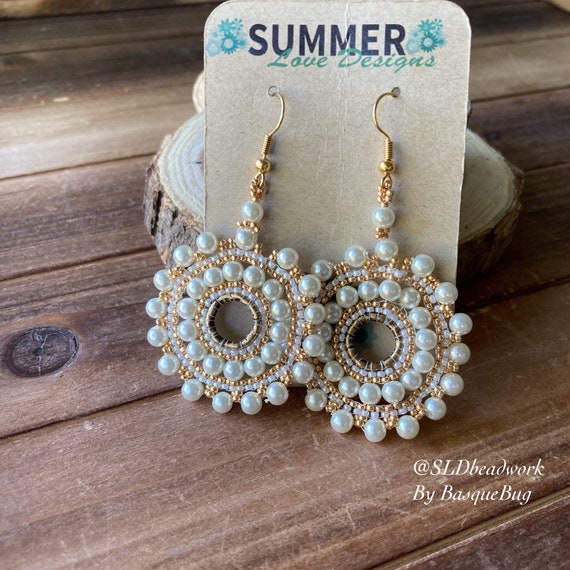The photograph displays a set of intricate, dangly earrings resting on a wooden table. The earrings are affixed to a brownish cardboard holder, leaning against a tree bark slice, giving it a rustic presentation. The cardboard plaque prominently features the words "Summer" in large black letters, followed by "Love Designs" in smaller green cursive letters, framed by bluish-green floral images. Each earring comprises a series of concentric circles, alternating between rows of pearls, white beads, and gold beads, with a distinctive central void that adds to their intricate design. The bottom right corner of the image contains the superimposed text "@SLDbeadwork" in black letters, with "by Bosque Bug" directly beneath it.